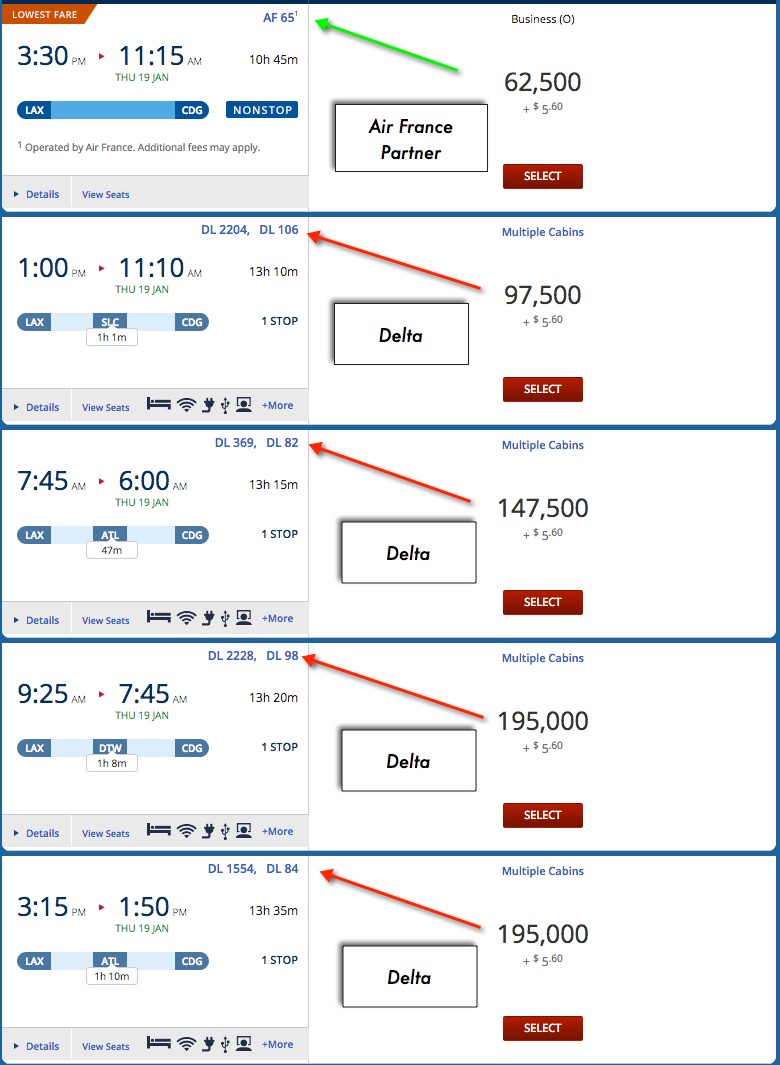This image is a screenshot from a website featuring a matrix of ten boxes arranged in two columns of five boxes each. Each box contains flight information with various color-coded tabs and bars. 

**Left-hand Column:**
1. **Top Box:** 
   - Upper-left corner: Green or orange tab labeled "Lowest Fare".
   - Below that: "3.30pm".
   - To the right: Red arrow pointing right, followed by "11.15am".
   - Centered below: Green text displaying "Thursday, 19 Jan".
   - Further below: Blue gradient bar transitioning from dark blue to light blue and back to dark blue.

2. **Second Box:**
   - "11pm".
   - Red arrow pointing right, followed by "11.10pm".
   - Below: Another blue bar.

3. **Third Box:**
   - "7.45am".
   - Red arrow pointing right, followed by "6.00am".

4. **Fourth Box:**
   - "9.25am".
   - Red arrow pointing right, followed by "7.45am".

5. **Bottom Box:**
   - "3.15pm".
   - Red arrow pointing right, followed by "1.15pm".

**Right-hand Column:** 
1. **Top Box:**
   - Across the top: Black-outlined white box labeled "Air France Partner".
   - Below: "62,500".
   - Bottom: Red bar labeled "Select" in white.

2. **Second Box:**
   - Top: White box labeled "Delta" in black.
   - To the right: "97,500".
   - Bottom: Red bar labeled "Select" in white.

3. **Third Box:**
   - Top: White box labeled "Delta" in black.
   - To the right: "147,500".
   - Bottom: Red bar labeled "Select" in white.

4. **Fourth Box:**
   - Top: White box labeled "Delta" in black.
   - To the right: "195,000".
   - Bottom: Red bar labeled "Select" in white.

5. **Bottom Box:**
   - Top: White box labeled "Delta" in black.
   - To the right: "195,000".
   - Bottom: Red bar labeled "Select" in white.

A consistent color scheme and layout are used across all boxes, punctuated by recurring visual elements such as red arrows, blue bars, and 'select' tabs, indicating flight options and their respective details.